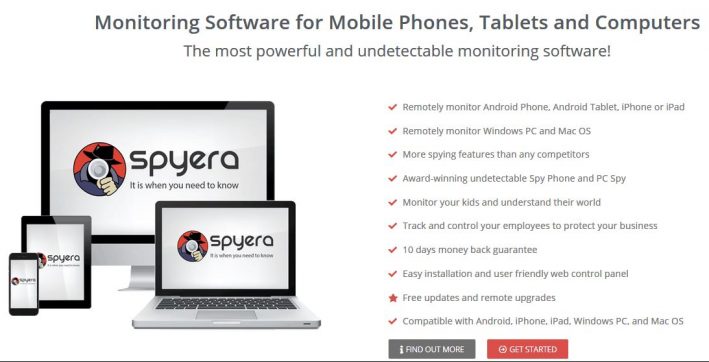The image features a block of text detailing the capabilities of advanced monitoring software for various electronic devices. The software is highlighted as the most powerful and undetectable in the market, designed to remotely monitor Android phones, Android tablets, iPhones, and iPads, as well as Windows PCs and Mac OS devices. It surpasses competitors in offering extensive spying features, ensuring comprehensive oversight both for parental control and employee monitoring. With an award-winning reputation, the software enables users to track and control online activities seamlessly, thus protecting family and business interests. Key highlights include a 10-day money-back guarantee, easy installation, a user-friendly web control panel, free updates, and remote upgrades. The text encourages potential users to find out more and get started. To the left of the text, the image also showcases various electronic gadgets such as smartphones, tablets, and laptops.